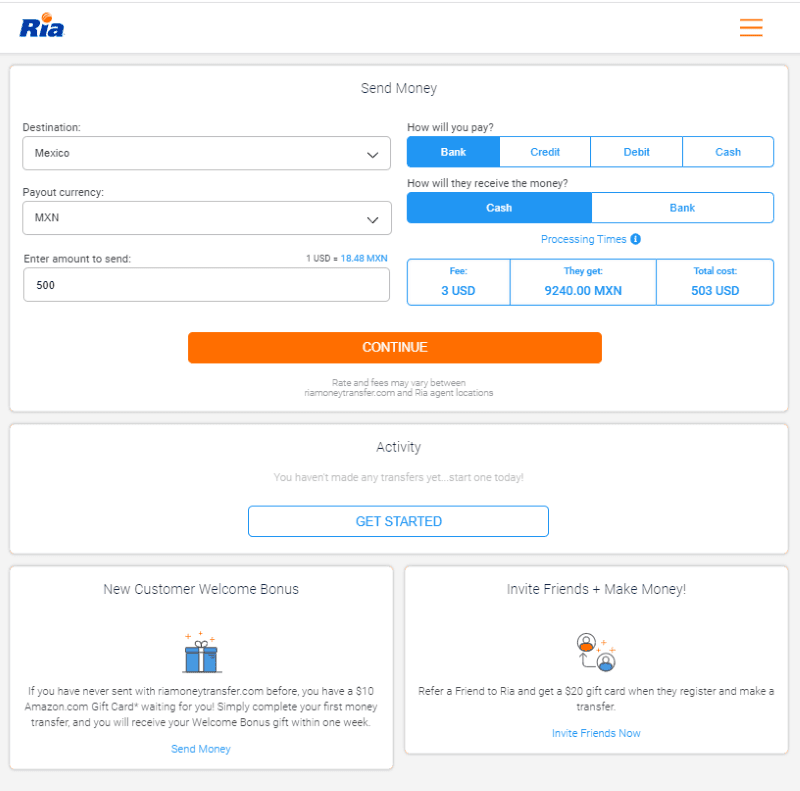**Website Screenshot Description: RIA Money Transfer Interface**

The captured webpage belongs to RIA Money Transfer and features their online money transfer interface. At the top, the site is branded with "RIA," where the I is creatively dotted with an orange dot. Adjacent to the logo are three parallel orange lines, likely serving as a menu or navigation indicator.

Below the header, there's a structured white box housing various text fields and menus which facilitate money transfers. The topmost heading "Send Money" is prominent in a combination of black and blue text. The interface allows for selecting the destination country with "Mexico" chosen, and the payout currency set to MXN (Mexican Pesos).

Specific options are visible for entering the transfer amount. The example displayed shows an input of 500 USD, automatically calculating the equivalent in MXN, which is approximately 18.48 MXN per USD. Instructions prompt users to specify the method of payment, indicated by four blue-highlighted options: "Bank" (selected), "Credit," "Debit," and "Cash."

Further down, users must select how the recipient will receive the money, with the options "Cash" (selected) and "Bank." Processing times are indicated with an "i" icon next to them, signifying additional information is available. Fee details are displayed in three boxes showcasing a $3 USD fee, resulting in the recipient receiving 9,240 MXN. The total cost is summarized as 503 USD. A prominent orange and white "Continue" button is available for proceeding with the transaction. A gray-font notice below advises that rates and fees may vary.

Scrolling down, a section labeled "Activity" states that no transfers have been made yet, inviting users to start one with a blue "Get Started" button.

Additional sections offer promotional information:

1. **New Customer Welcome Bonus:**  
   Features a blue gift box icon, encouraging new users to make their first transfer, promising a $10 Amazon.com gift card within one week as a welcome bonus.
  
2. **Invite Friends + Make Money:**  
   Displays icons of two cartoon people (one orange, one blue), offering a $20 gift card for referring friends who register and make a transfer. A blue "Invite Friends Now" link facilitates this referral process.